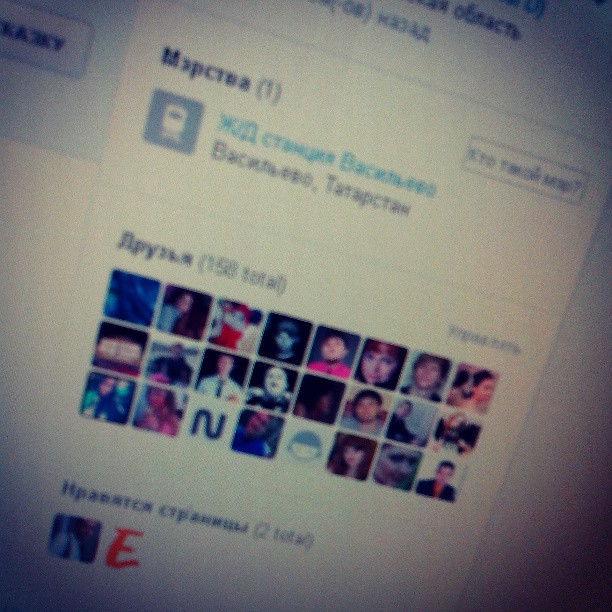This image appears to be a grainy, blurred photo of a social media website page written in a foreign language, likely Russian or Croatian. The language barrier is evident as the text at the top is unreadable, but there is a noticeable section with blue text followed by a number in parentheses. Central to the image are 24 small, square thumbnails arranged in a grid of three rows, each displaying eight images. These thumbnails include a mix of human faces, emojis, and a blue letter "N," likely representing the user's friends on the site. Adjacent to this grid, there is a heading with a foreign word and "158 total" in parentheses, indicating the total number of friends. At the very bottom right of the page, another section is mentioned with "two total," featuring a red "E" and a blurred image, potentially an advertisement. The photo itself appears to have a dark, high-contrast filter applied, giving it a vignetted look.